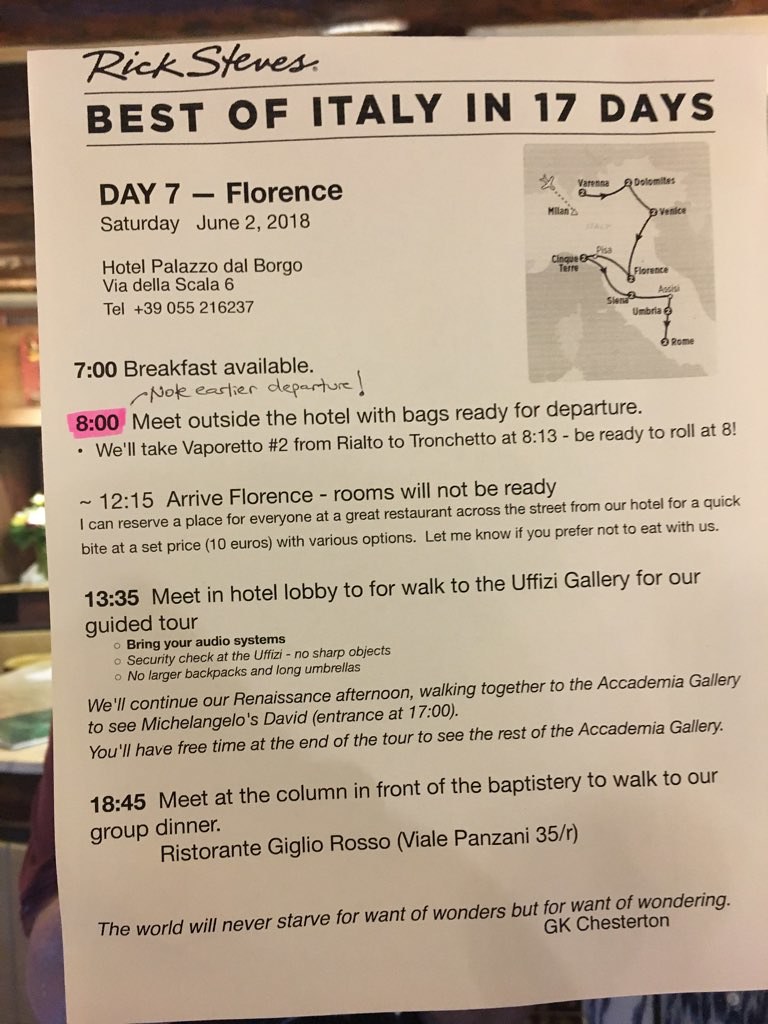This image is a clear, printed itinerary on a light beige piece of paper for a structured tour by Rick Steves, highlighting the "Best of Italy in 17 Days." It focuses on Day 7 in Florence, scheduled for Saturday, June 2, 2018. The itinerary includes detailed timings and activities:

- **7:00 AM:** Breakfast available.
- **8:00 AM:** Meet outside the Hotel Palazzo Dal Borgo, via Della Scala 6, with bags ready for departure. No early departures noted. 
- **8:13 AM:** Take Vaporetto No. 2 from Rialto to Tronchetto.
- **12:15 PM:** Arrive in Florence; rooms will not be immediately ready. Optional lunch at a restaurant across the street from the hotel for a set price (10 euros), with varied menu options.
- **1:35 PM:** Meet in the hotel lobby for a walk to the Uffizi Gallery for a guided tour. Important instructions include bringing your audio system and being prepared for security checks—no sharp objects, large backpacks, or long umbrellas.
- **After Uffizi:** Continue the Renaissance tour to the Accademia Gallery to see Michelangelo's David, with entry at 5:00 PM. Free time will be provided afterwards to explore the rest of the gallery.
- **6:45 PM:** Meet at the column in front of the Baptistery to walk to the group dinner at Ristorante Giglio Rosso.

The paper also features a motivational quote by G.K. Chesterton: "The world will never starve for want of wonders, but for want of wondering." There is a small map in the upper right corner showing the tour's route across Italy. The paper includes the hotel's contact number: +39-055-216-237.